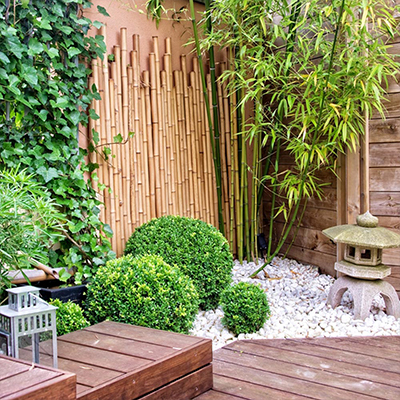This is an outdoor photograph showcasing a serene Japanese garden. In the foreground, there's a dark brown wooden deck that leads to a carefully arranged patch of white pebbles. Scattered among the pebbles are three small, short bushes, and on the right side, a stone statue resembling a traditional Japanese lantern or pagoda with an overhanging roof adds an authentic touch. Climbing up the left side of the image is a lush cascade of ivy or vines. Central to the layout and creating a backdrop are bamboo stalks both laid against and growing out from what appears to be a wooden fence made of weathered, horizontal slats. The overall scene is a harmonious blend of natural elements and traditional Japanese garden features, creating a tranquil space.